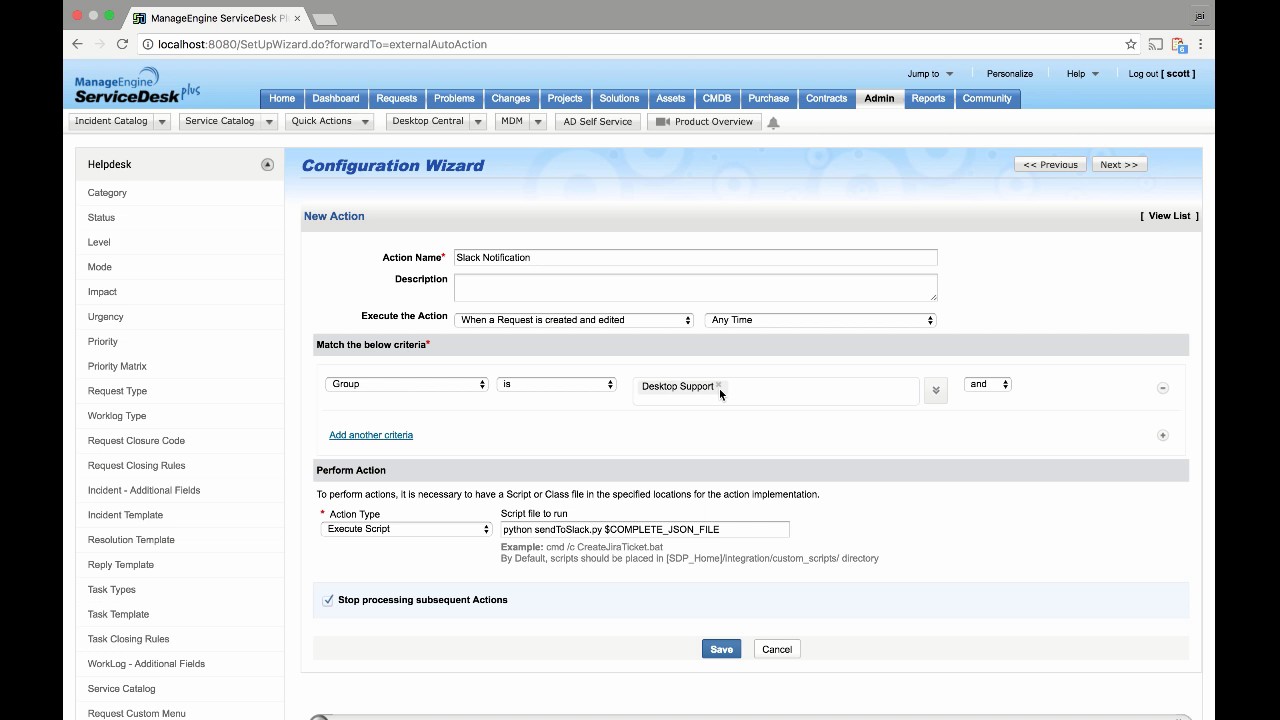The image depicts a dashboard interface featuring a multitude of sections and functionalities. In the top left corner, text in red, grey, and green backgrounds labels sections such as "Manage Engine" and "Service Test". A prominent area displays the text "localhost:8080/setupwizard.to", indicating a link to a setup wizard, which appears to forward to an external auto action related to "Manage Engine" and "Service Test". The interface is predominantly blue, with clearly defined areas for navigation including "Home", "Dashboard", "Request", "Problems", "Projects", "Deletions", "Assets", "CMDB", "Purchase", "Contracts", "Admin", "Reports", "Community", "Instant Catalog", "Service Catalog", "Quick Action", "Desktop Central", "MDM", "AT", "Subservice", "Product Overview", and "Configuration Wizard". There are fields for "Action", "Action Names", "Documentation", "Description", and options to "Execute the Action" when requests are created at any time, with conditions to match specific criteria. The interface includes various types of text, aiding navigation and functionality descriptions throughout.